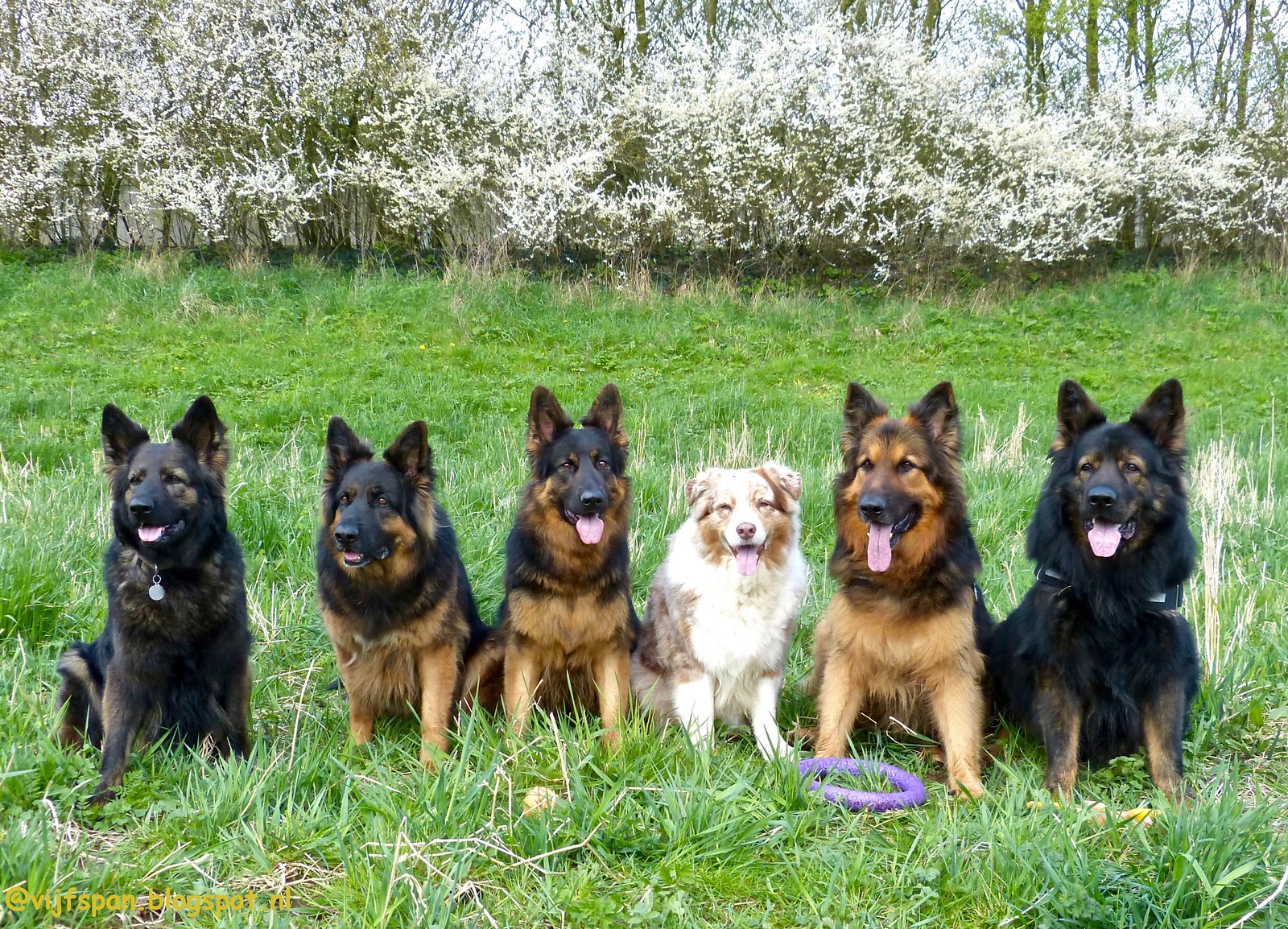In this picturesque scene, we see six dogs seated shoulder to shoulder in a lush, unmown grassy meadow, with tall green weeds and trees adorned with delicate white blossoms framing the background. Among the dogs, five are German Shepherds with varying coat patterns: two are nearly entirely black with slight brown markings around their eyes and legs, while the other three display the traditional German Shepherd coloring of brown and black with distinctive black masks. Nestled in the middle is a smaller dog with a strikingly different appearance, characterized by light gray and white fur with some brown around its face and a white streak running up its nose. This dog stands out not only because of its color but also its fluffy texture. One of the German Shepherds has a chew toy, a Frisbee-like tossing ring, placed in front of it, adding a playful touch to this serene outdoor tableau.